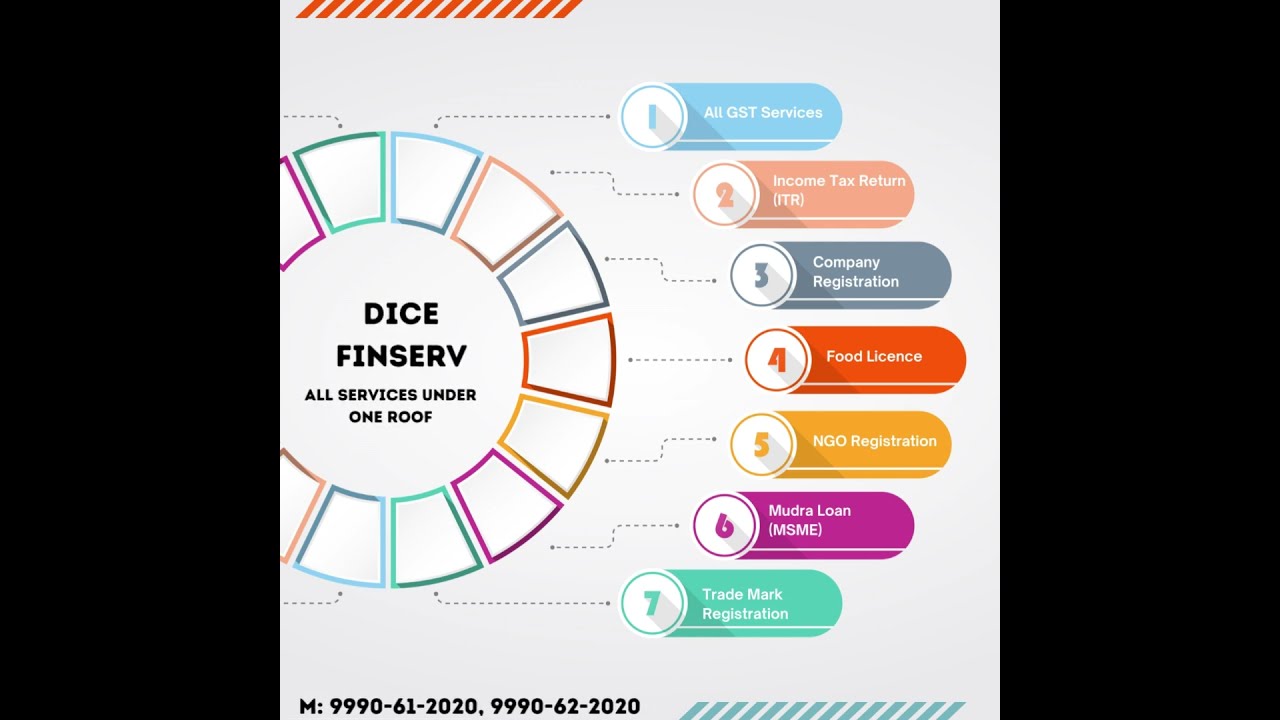The image is a color infographic set within a landscape-oriented black frame. The infographic itself has a square format with a light grey background. In the upper left corner, there's an orange stripe. Below this stripe, a circular color wheel is positioned at the center-left of the image. This wheel features various pie-shaped segments in colors such as green, blue, orange, dark green, red, yellow, and turquoise. Central text within the wheel reads "DICE FinServ" and "All services under one roof" in black letters.

To the right of the color wheel, there are seven multicolored rounded rectangles, each containing white text and numbered 1 to 7. Each rectangle corresponds to a segment of the wheel, with colors matching the segments and arrows connecting them. The bullet points in these rectangles are:

1. All GST Services
2. Income Tax Return (ITR)
3. Company Registration
4. Food License
5. NGO Registration
6. Mudra Loan (MSME)
7. Trademark Registration

In the lower left corner, there is text resembling a phone number: "M: 9990-61-2020, 9990-62-2020." The illustration includes an orange hash-like barcode at the top and a blue turquoise stripe at the bottom right corner. 

The infographic has a consistent graphic representational style, effectively outlining the various services offered by DICE FinServ.